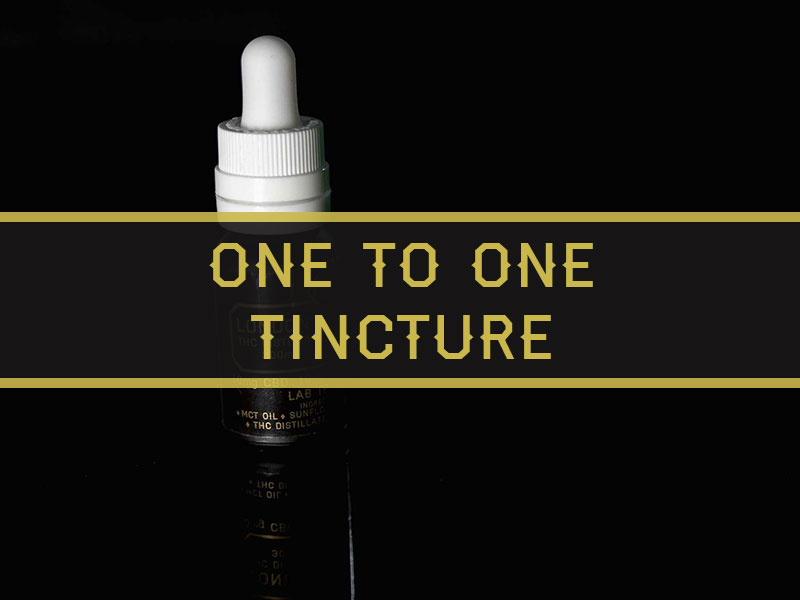The advertisement features a strikingly dark and severe image, dominated by a black background that accentuates a central dropper bottle. The bottle has a distinctive black lower half and a white rubber squeeze tip, resembling a baby's binky. Overlaid in the middle of the image is a black banner bounded by gold horizontal lines and text, which obscure part of the bottle's label. The gold text on the banner reads "one-to-one tincture." Gold lettering on the bottle itself mentions "MCT oil" and "THC distillery," although much of the detail is hidden by the banner. The overall design compels viewers to focus on the sleekly styled bottle amidst the otherwise minimalist and dark setting.